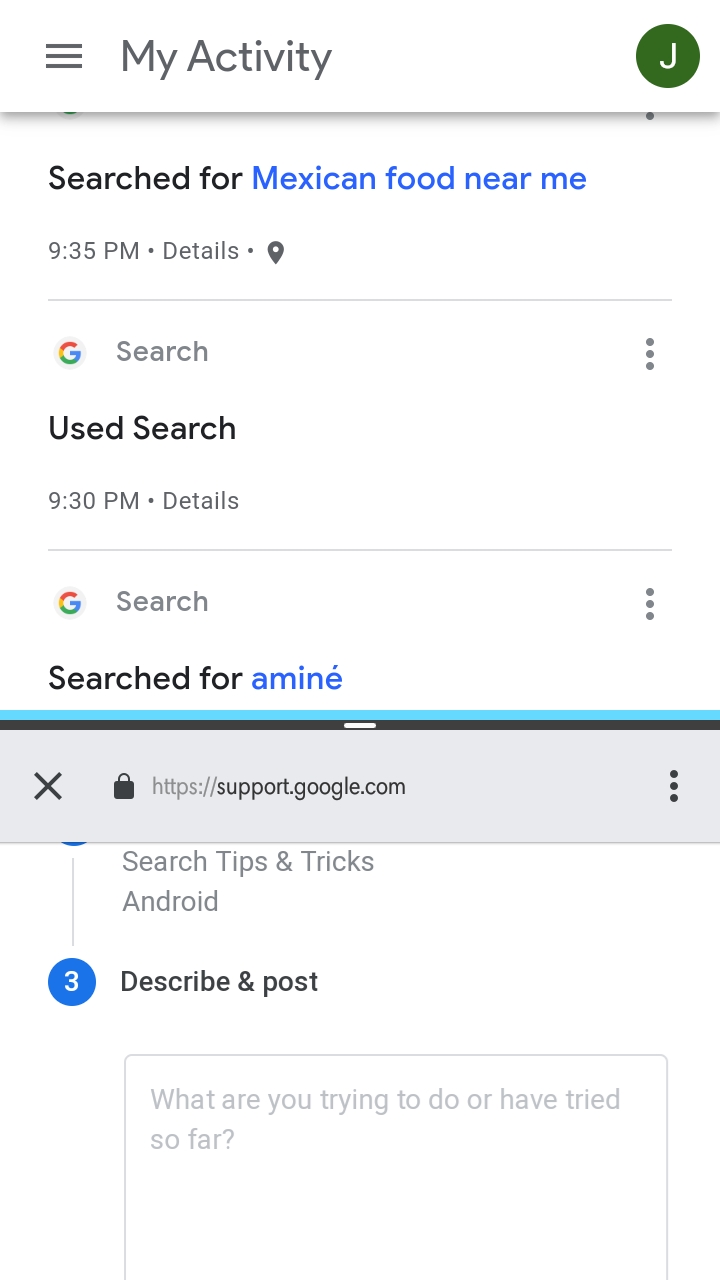The image is a smartphone screenshot with a white background, showcasing the "My Activity" page from Google. At the top left, a gray "My Activity" title appears beside a trio of horizontal gray lines, indicating a menu. On the upper right corner, a green circle with a white letter "J" serves as the user's profile icon.

Below the "My Activity" header, there's a gray dividing line. Under this line, the entry "searched for Mexican food near me" in blue font is timestamped at 9:35 PM, accompanied by a gray "Details" link and a small gray location icon.

The subsequent entry is labeled "Search" and features the multi-colored Google "G" logo. It states "used search" at 9:30 PM, also followed by a gray "Details" link.

Further down, another "Search" entry reveals a query "searched for anime," with "anime" spelled in blue font including an accented "é." Below this, a gray rectangle contains a gray padlock icon, indicating a secure website, alongside the support.google.com address. 

Next, in gray text against the white background, are the words "Search tips and tricks Android." Underneath, a blue circle with the number "3" in white is displayed next to the phrase "describe and post." Nearby, a lightly outlined gray box contains the light gray placeholder text, "What are you trying to do or have tried so far?"